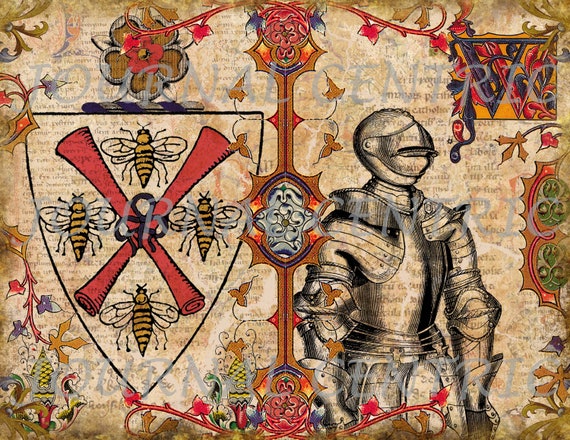The image is a highly intricate and colorful tapestry-style artwork, possibly from the medieval period. It is divided into two halves. On the left side, there is a detailed coat of arms. This shield prominently features a red X made from two rolled-up scrolls, with each quarter of the X containing a honeybee. Surrounding the shield are ornate designs in several bright colors, adding to its complexity. 

On the right half of the artwork stands a suit of armor, fully covering a man from head to hips, though no facial features are visible. Above this figure, in the upper right corner, is a beautifully crafted letter 'W' in dark blue, silver, and red. The entire scene is bordered with intricate patterns of flowers and shapes, contributing to its detailed appearance.

The background of the artwork includes barely readable texts resembling newspaper prints, adding a layer of depth and texture. The predominant colors throughout the piece are brown, red, and gold on a pale cream-brown background, which ties together the entire mural with an elegant, historical feel.